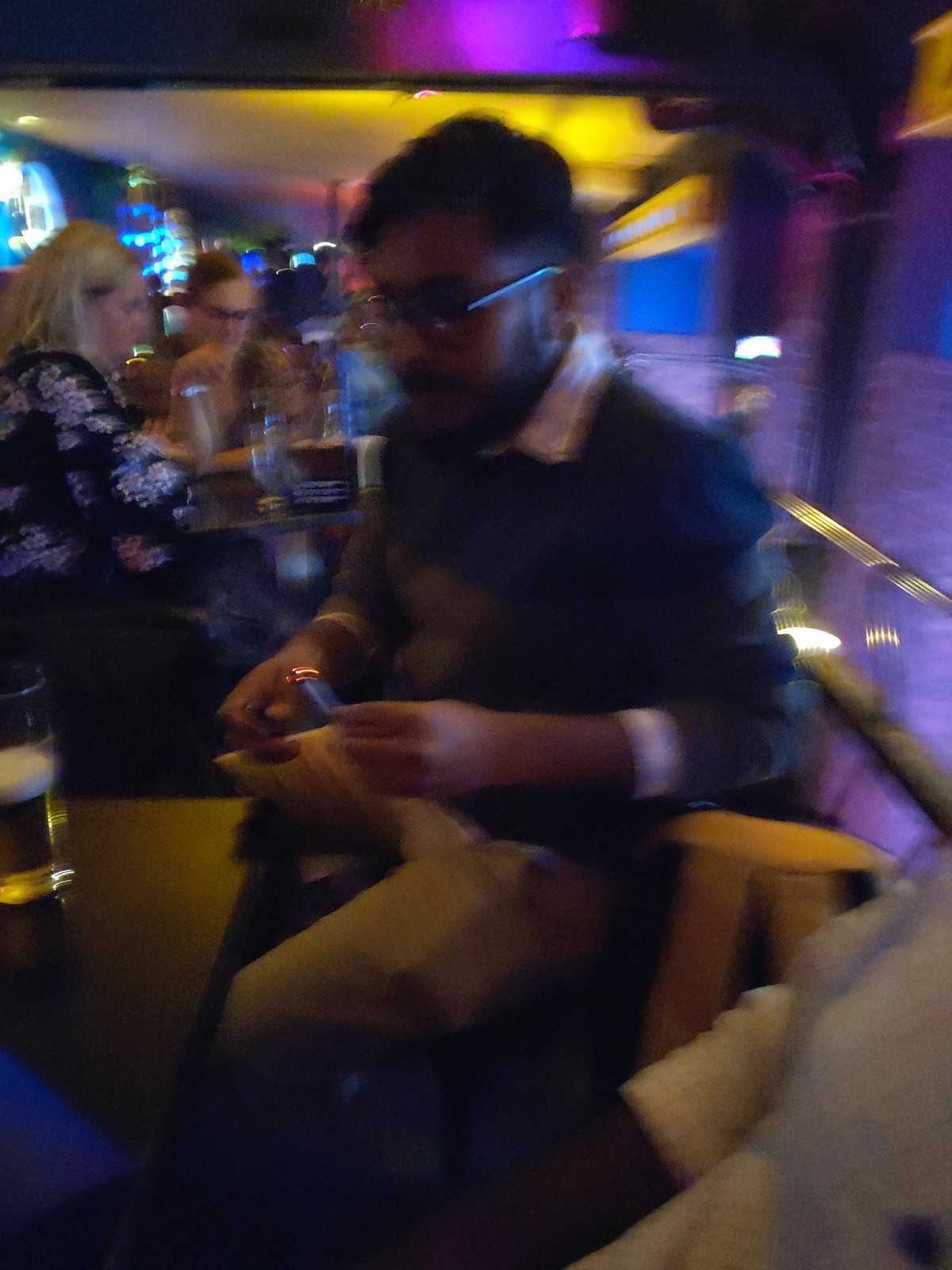Despite the low quality and blurry nature of the image, certain details are distinguishable. At the center of the image, a man with black hair and glasses is seated. He has a mustache and a beard, and he is dressed in a blue shirt over a white-collared inner shirt. His tan-colored pants are also visible. The man is holding an indeterminate object in his left hand due to the blurriness. To the man's left stands a table with a glass filled with a yellow liquid on it.